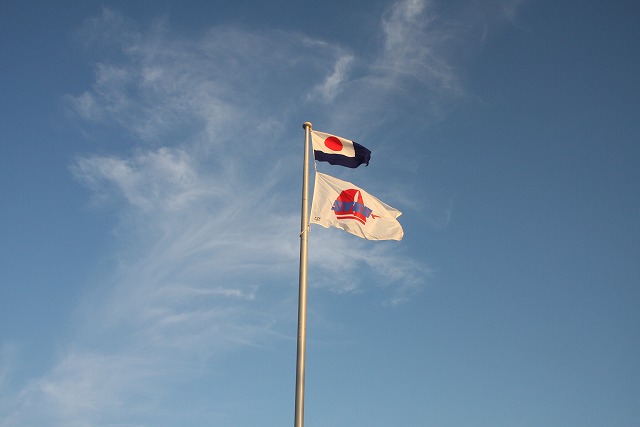The image captures a low-angle shot of a silver flagpole standing starkly against a clear blue sky dotted with wispy, white clouds. The flagpole is adorned with two flags, both rippling in the wind. The top flag closely resembles the Japanese flag, featuring a prominent red circle at its center set against a white background, but it is bordered with blue, suggesting it might not be the exact national flag of Japan. Below it, a second white flag is visible, marked by a red illustration of a sailboat and some blue text, the lettering of which begins with an "S" but remains largely indecipherable due to the image resolution. The scene is devoid of any other features or landmarks, emphasizing the vibrant movement of the flags against the serene day sky.